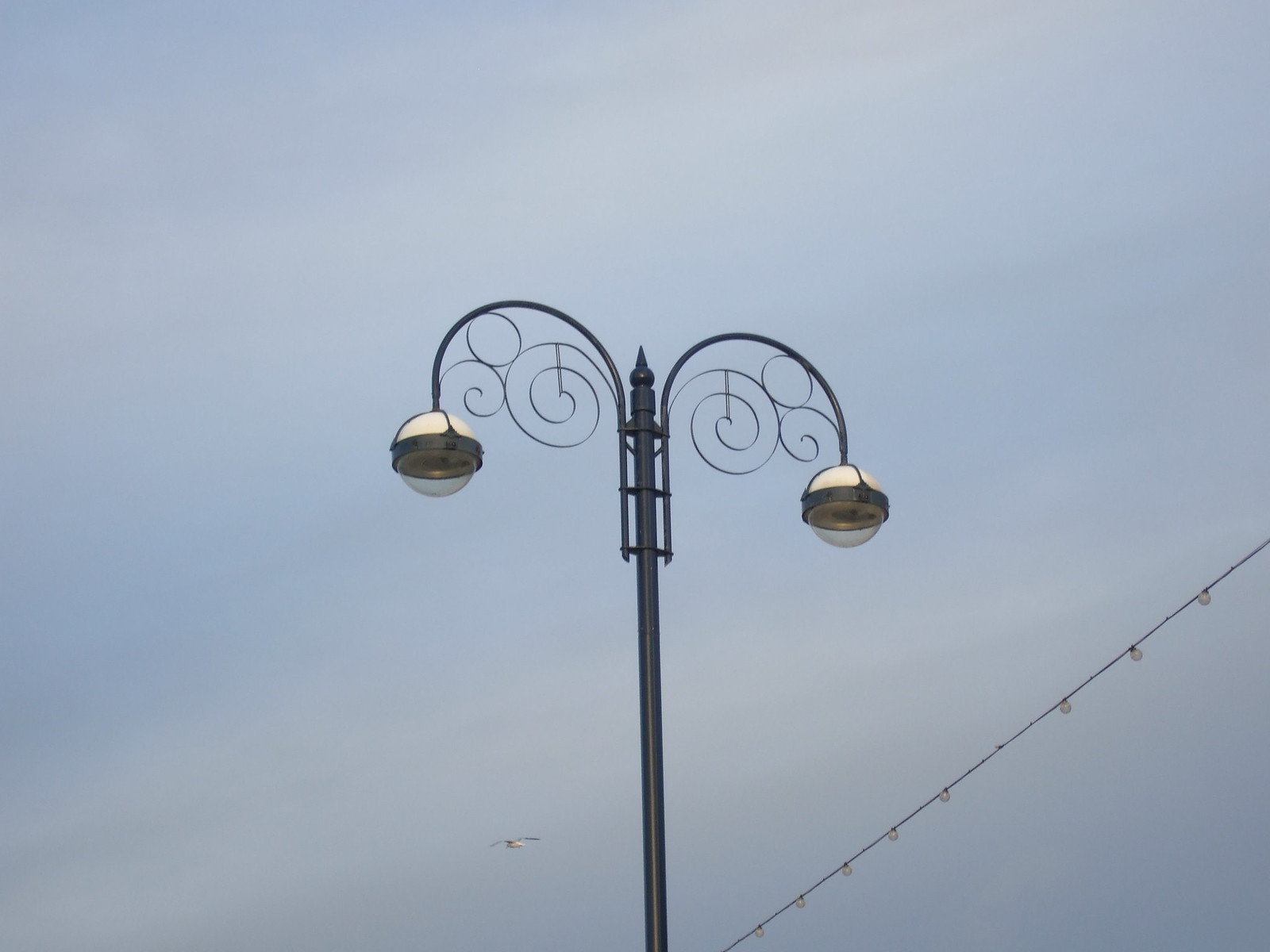The image presents a detailed view of an elegantly stylized bluish lamppost against a backdrop of a pale grayish-blue sky with subtle white hazy clouds. The lamppost, artistically designed, features two curved metal arches extending from the center, each adorned with intricate swirling patterns. At the end of these arches hang spherical lamps framed in blue with white tops and transparent covers, allowing light to filter through. Below, on the left side of the lamppost, a small bird can be seen in flight, while a string of outdoor bulbs stretches across the bottom right corner, adding to the outdoor ambiance. This carefully composed image captures the graceful architecture of the lamppost as it rises against the serene daytime sky.